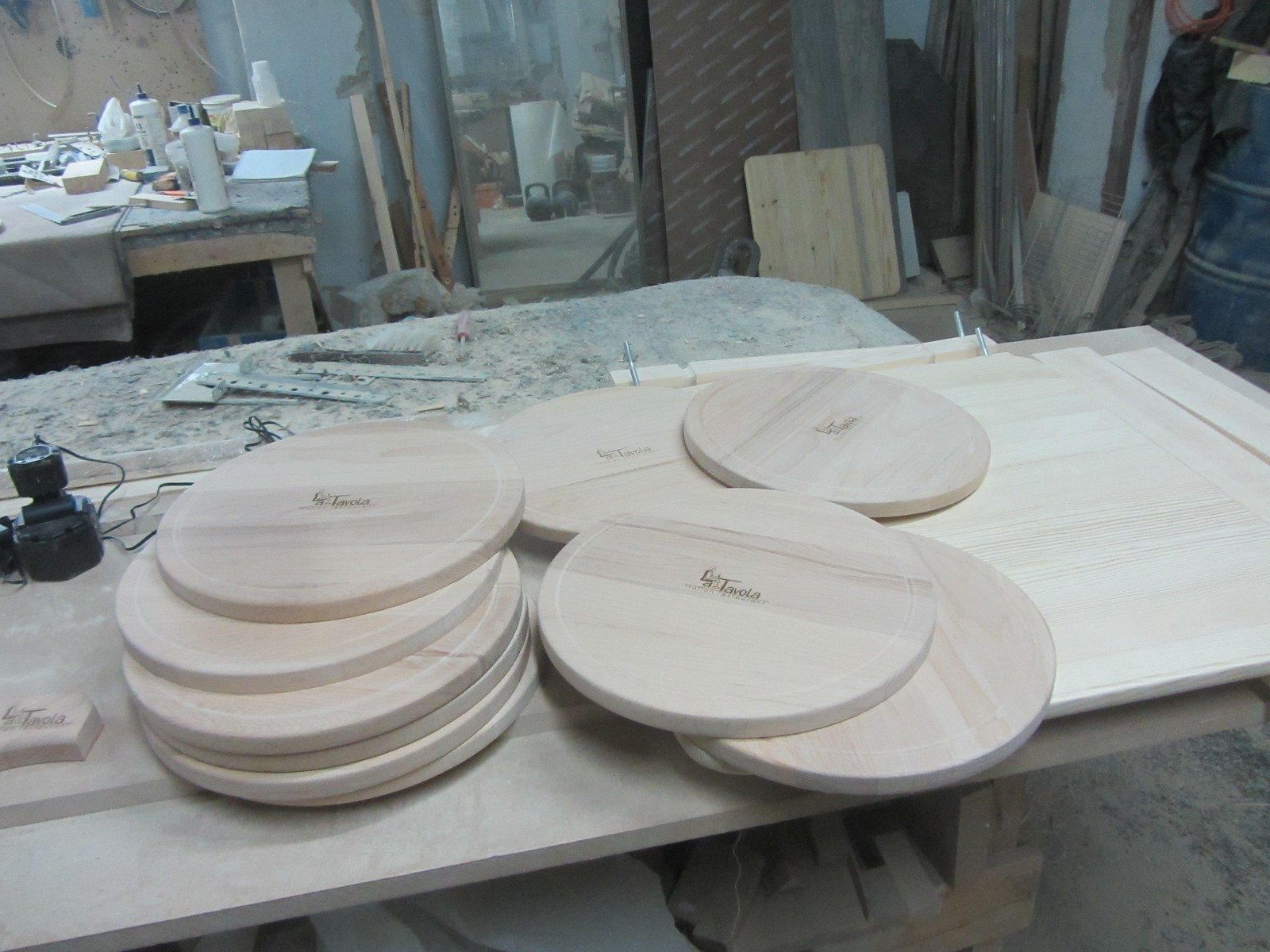In this photograph of a woodworking workshop, wooden discs—likely coasters—are prominently displayed on a surface cluttered with wood shavings, dust, and a variety of tools. These discs have been meticulously cut, sanded, and branded with the text "LA TAVOLA," though the finer details of the branding are somewhat blurred. The surface appears to be either stone or heavily marked with woodworking residues, and behind it, additional workbenches are visible. These benches hold rulers, a T-square, electronic measuring devices, and sandpapered, dust-coated tools, including a rust-coated screwdriver with a red handle. Various woodworking planes and tall white bottles of wood glue are also present. The workshop has a rustic atmosphere, with barrels and stacked wood pieces scattered across the floor, ready for future projects. A mirror leans against the wall, reflecting parts of the room and adding to the sense of depth in this busy and functional space dedicated to crafting small wooden items for sale.